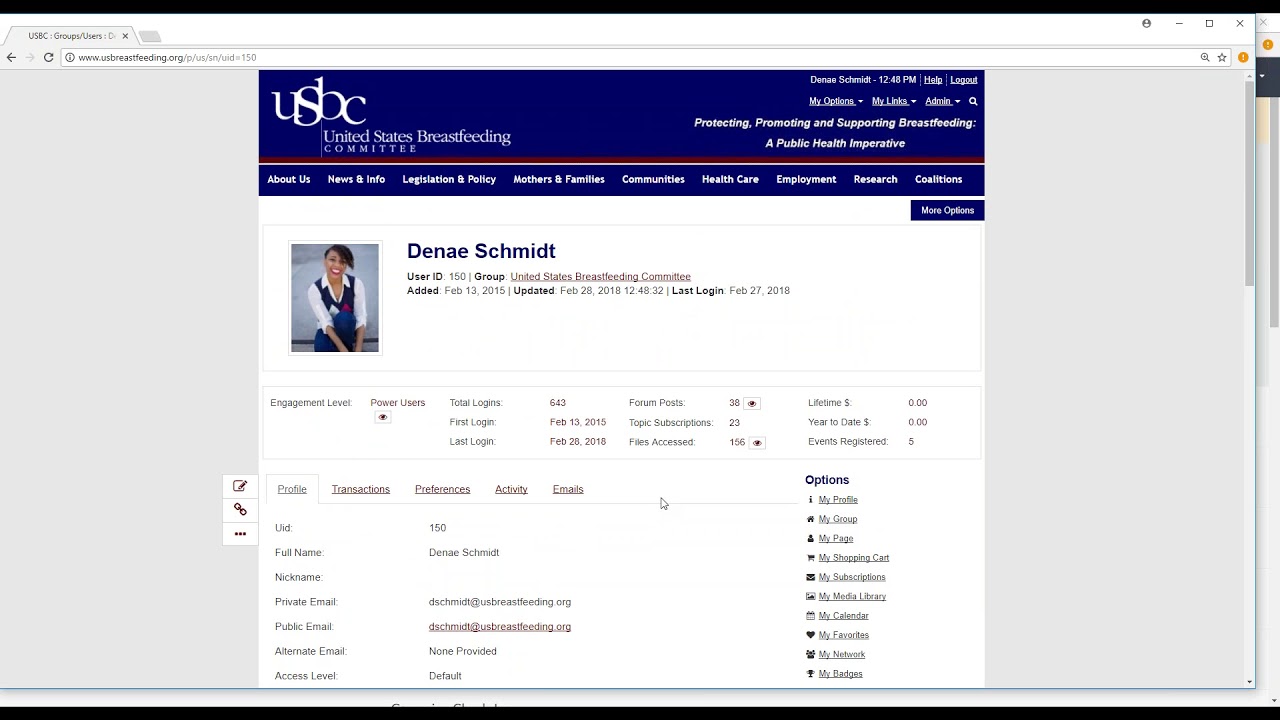In the image, a browser window is open with a tab displaying the website usbreastfeeding.org, which features a blue header. The header prominently displays "USBC, United States Breastfeeding Committee." On the right side under the header bar, the name "Dina Schmidt" is shown along with the timestamp "12:48 PM" and navigation options such as "Help," "Logout," "My Options," "My Links," "Admin," and "Search." Below the header, a tagline reads, "Protecting, promoting, and supporting breastfeeding, a public health imperative." This is followed by a red line and a white line, above a navigation menu with items in blue and white text: "About Us," "News and Info," "Legislation and Policy," "Mothers and Families," "Communities," "Healthcare," "Employment," "Research," and "Coalitions." A small blue button labeled "More Options" is also visible. The profile information for Dina Schmidt includes a user ID of 150, associated group "United States Breastfeeding Committee," and details that the profile was added on February 13, 2015, and last updated on February 28, 2018, at 12:48 PM, with the most recent login on February 27, 2018. Engagement level is marked as "Power User," with a total of 643 logins.